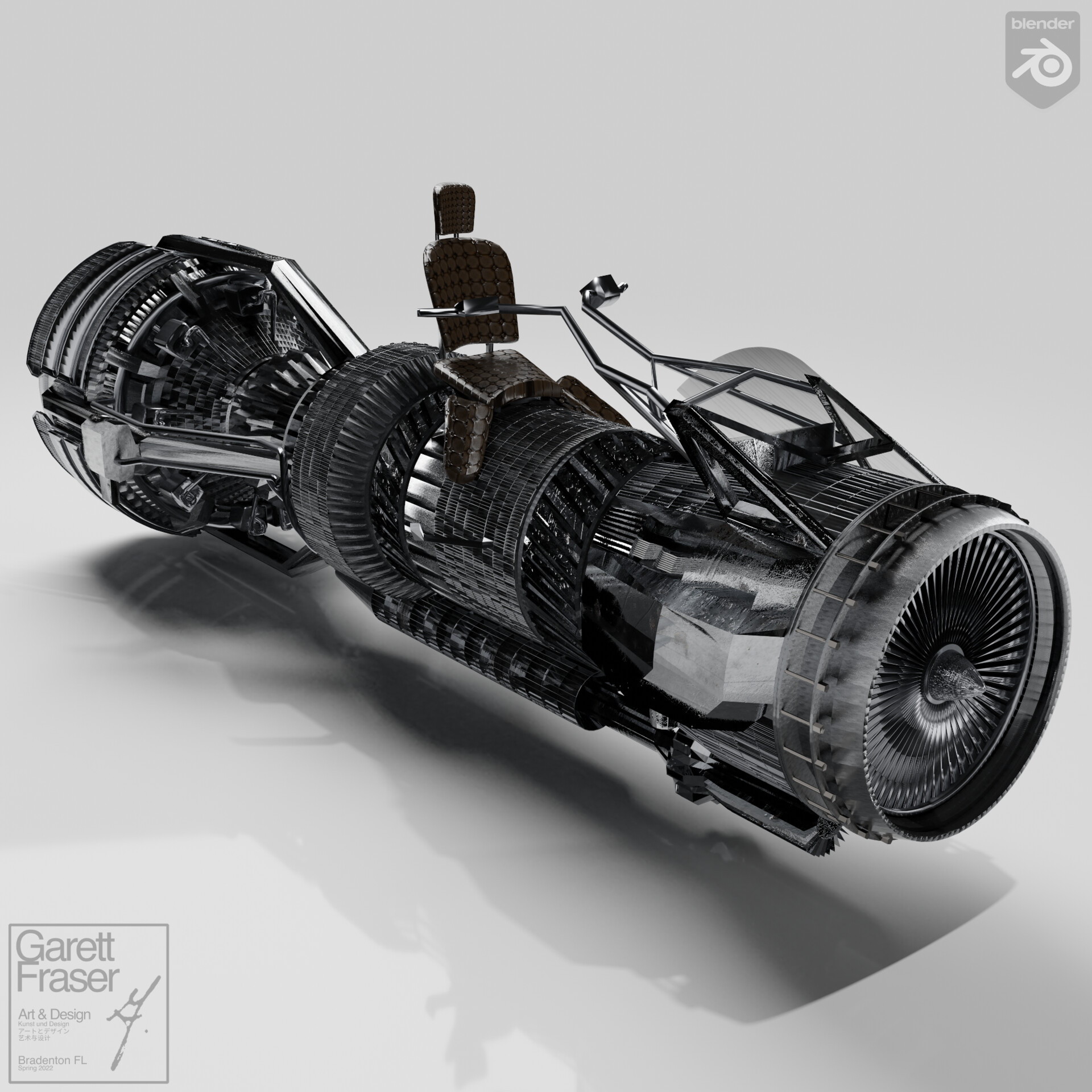The image showcases a sleek, all-black futuristic object with silver accents, resembling a cross between a motorcycle and a hovercraft. Set against a grey background, the design seems highly technological, featuring a chair on top and handlebars in the front, suggesting it can be ridden like a motorbike. The object incorporates multiple connected fans, with the largest one positioned at the rear, likely providing propulsion. There's a vent at the front, indicating an engine or fan mechanism. The lower left corner of the image contains the text "Garrett Frazier, Art and Design in Bradenton, Florida," identifying Garrett Frazier as the artist. In the upper right corner, the word "Blender" appears alongside its emblem, a circle with three lines emanating from it.